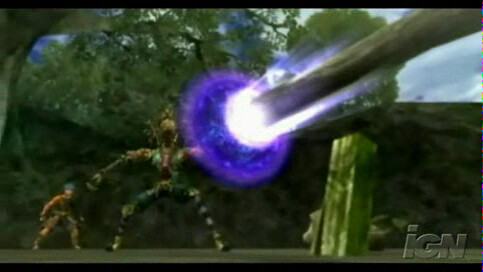In this widescreen image from a video game, a warrior stands in a defensive stance in the foreground. The bottom right corner features a watermark with "iGN," where the 'i' is lowercase and the 'G' and 'N' are uppercase. The warrior, a fantastical creature distinguished by its humanoid form with clear arms, legs, torso, and head, is grasping a shield in its left hand. Vibrant beams of light, indicative of a laser or light-based attack, reflect off the shield, suggesting an intense confrontation. Behind the shield-bearing warrior, another creature, seemingly unprotected and vulnerable, seeks shelter, indicating that the warrior is actively defending its comrade from the oncoming assault.